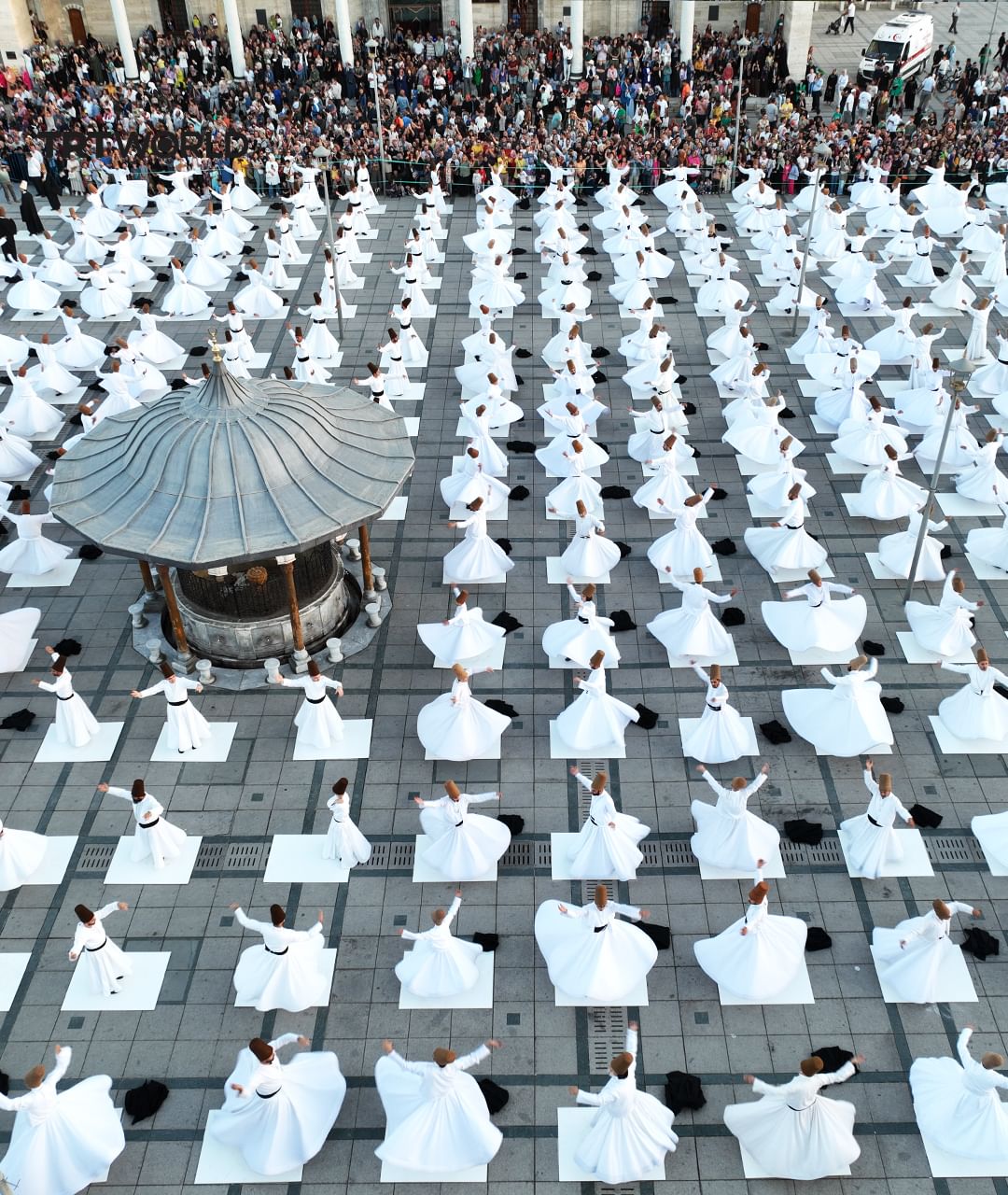This overhead photograph captures a bustling city square, predominantly paved with silver and gray blocks. At its center, a large group of women dressed in ankle-length white dresses are arranged on white mats, appearing to perform a dance routine with their hands lifted in the air, causing their dresses to flare out. The scene is lively, with at least forty to fifty performers spaced evenly across the patterned ground. On the left side of the image stands a small, pavilion-like structure with a gray, circular roof. The background reveals a dense crowd, held back by ropes, eagerly watching the performance. Dominating the palette of the photograph are shades of silver, gray, and white, with occasional details such as dark brown and black hair visible among the dancers. At the top-left corner, there is a watermark or logo, reading "TRT World" in brown text. The overall ambiance suggests a significant and coordinated public event, captured during daylight.